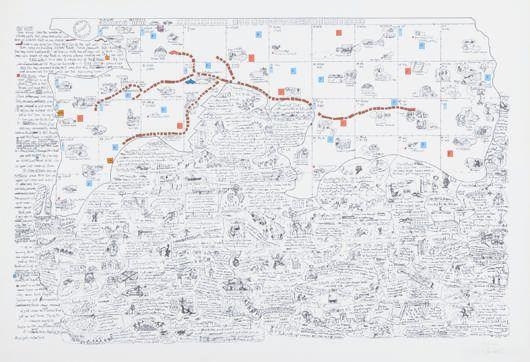This image depicts an intricate and unconventional map, not representing a world or country map. The rectangular-shaped map is rich in detailed text and various icons, although the text remains difficult to read. A prominent pathway of interconnected lines created with red-colored dots traverses the map. The rest of the map predominantly features a black and white color scheme, accentuated with some colored dots in orange and blue. Certain areas are marked with colorful boxes, possibly red and blue, adding to the complexity of the design. The map's outline is thin and black, resembling the shape of a state, potentially Kansas, and overall, it gives the impression of a vintage or storybook illustration.